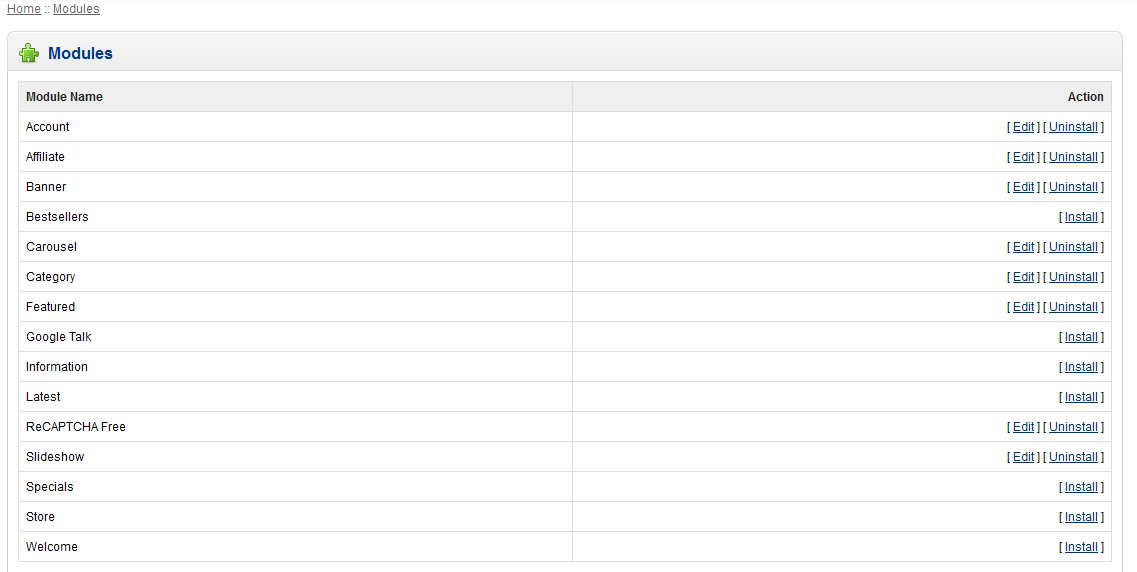The image depicts a webpage from a website, showcasing a specific section dedicated to modules. The interface includes a navigation menu at the top with 'Home' and 'Modules' options, where the 'Modules' section is currently open. The overall design primarily uses a navy blue and green color scheme, with a gray background. The word 'Modules' is prominently displayed in a bluish navy color adjacent to a green puzzle piece icon, symbolizing the module components.

The page layout is divided into two main columns by a faint gray line. The left column lists module names, while the right column contains action links for each module. These clickable links are labeled in blue and offer options such as 'Edit', 'Install', 'Uninstall', and combinations thereof. The detailed module list under 'Module Name' includes:

1. Account
2. Affiliate
3. Banner
4. Bestsellers
5. Carousel
6. Category
7. Featured
8. Google Talk
9. Information
10. Latest
11. Recaptcha Free
12. Slideshow
13. Specials
14. Store
15. Welcome

Each module name is separated by a faint gray line, creating a structured and organized view.